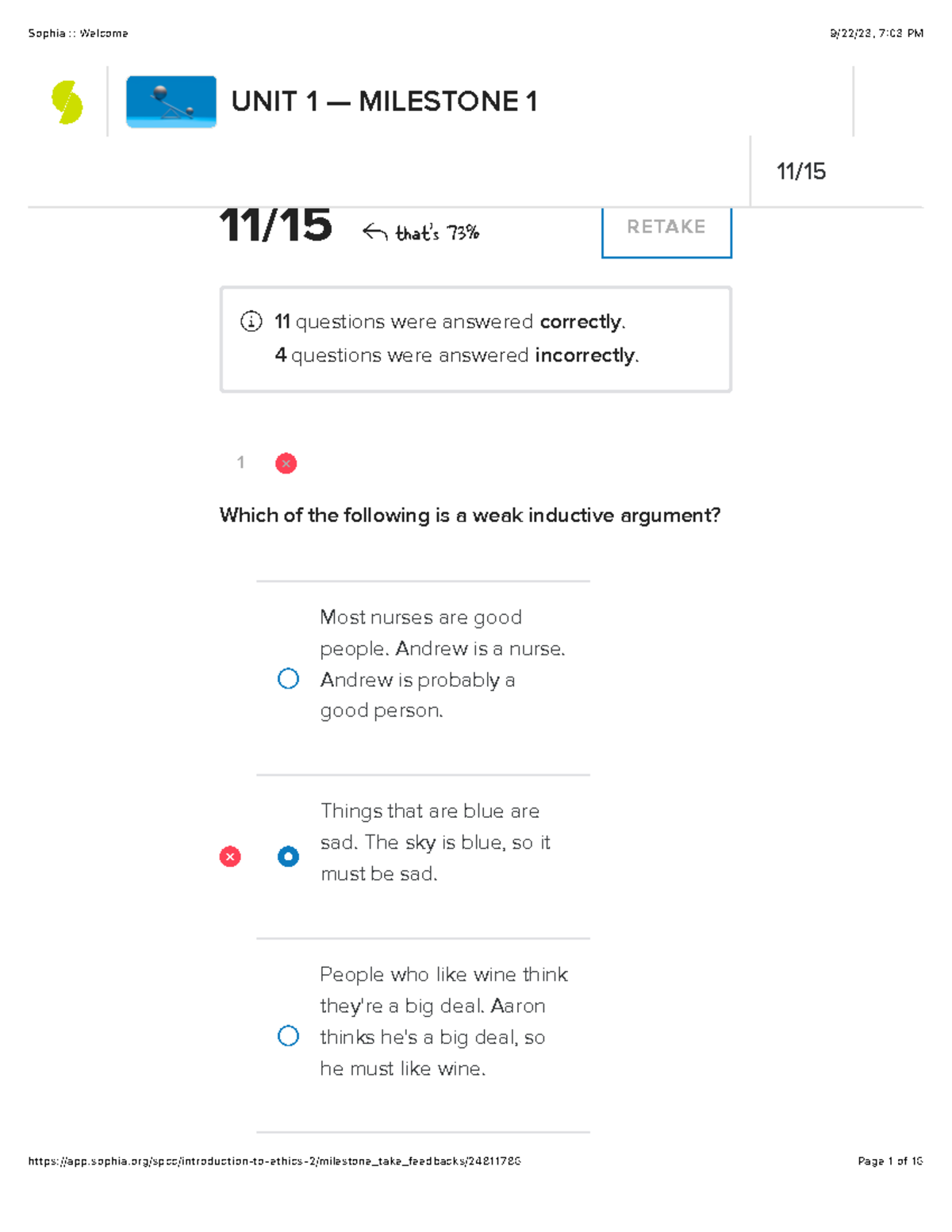In the image, the top left corner displays information related to Sophia's progress on "Unit 1, Milestone 1." Sophia scored 73%, correctly answering 11 out of 15 questions, with 4 incorrect answers. Additionally, the section poses a question: "Which of the following is a weak inductive argument?" Three choices are listed:
1. "Most nurses are good people. Andrew is a nurse. Andrew is probably a good person."
2. "Things that are blue are sad. The sky is blue, so it must be sad."
3. "People who like wine think they are a big deal. Aaron thinks he is a big deal, so he must like wine."

Below this information, there is a noticeable link, though its destination is not specified in the description. 

In the bottom right corner of the image, it indicates that this is "Page 1 of 16," suggesting there are additional pages of content.